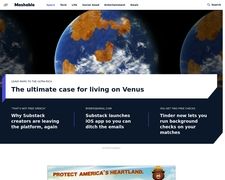The image depicts an article page, although much of the text appears blurred. The visible headline prominently reads, "The Ultimate Case for Living on Venus." Accompanying the article are illustrations or images of planets, adding a visually engaging element to the page. At the bottom of the page, another piece of visible text states, "Protect America's Heartland." The combination of these elements suggests a discussion on space exploration or habitation, possibly juxtaposed with themes of environmental or national protection.